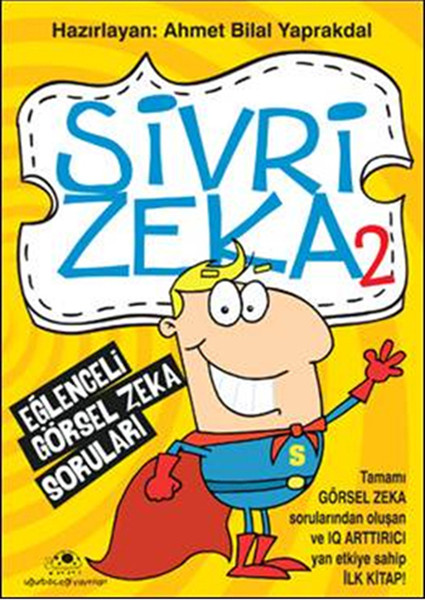The image appears to be a vibrant comic book or children's book cover in a foreign language, featuring a cartoon superhero. The top of the cover displays large blue text reading "Sirvizika II." Below this title, there's a cartoon depiction of a boy with blonde hair, wide eyes, and big teeth. The superhero is dressed in a blue costume with a yellow "S" on the chest, complemented by a red cape, red gloves, red boots, and a blue belt with a yellow buckle. He is smiling and waving towards the viewer. The background consists of swirling yellow and darker yellow circles. Additional text in the image includes "Hazelayan Amet Bilal Yaprakdal" at the top, "Inglisir Gorsel Zika Zorluari" in black boxes with white letters to the left of the superhero, and "Tamami Gorsel Zika Sorrendenlusen V.I.Q. Atresiyan Etika Sahip Ilkitap!" in smaller letters to the bottom right. A small ladybug icon appears in the bottom left corner. Overall, the cover has the aesthetic of a comic book or a children’s book, characterized by its bold colors and playful design.